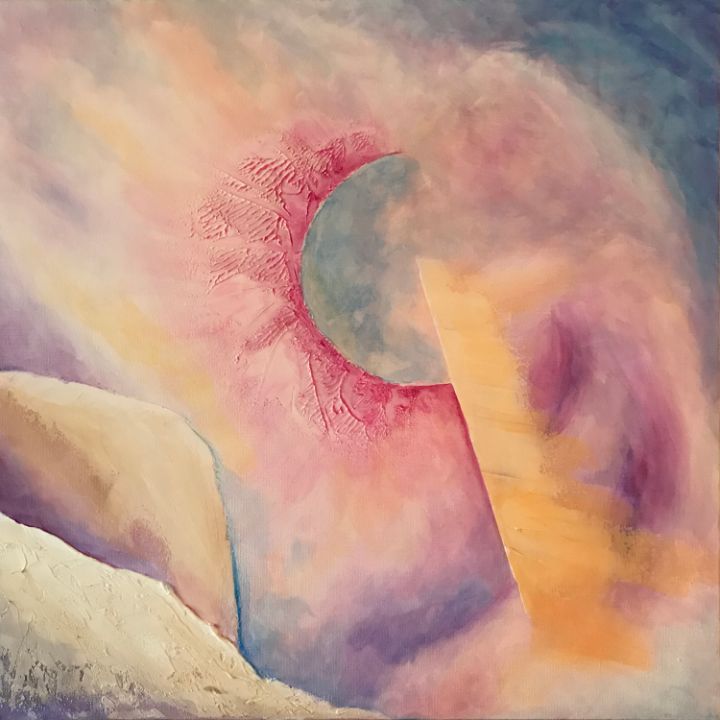This image is an abstract painting possibly executed in oil. The dominant feature is a partial circular form that could represent a sun or moon, set against a textured blue background. Surrounding this circle are vibrant red smudges and flares in various textures and hues, including yellow, orange, and pink. In the upper right corner, the dark blue sky, tinged with cream and gray, suggests an atmospheric quality. The sun or moon figure itself is a mix of green, blue, and yellow tones, interspersed with purple spheres and textured elements. A diagonal green bar cuts across the composition from the bottom right to the top center. The left-hand corner of the painting features large gray boulders, one situated on an incline, the other being more rectangular. An overlay of dreamy, mushed colors creates a foreground that might be interpreted as white hillsides or rocky terrains. The top right corner features a notable dark surface, adding depth and contrast to the scene, which can be imagined as a sun obscured by clouds and rocks in a surreal, abstract outdoor setting.